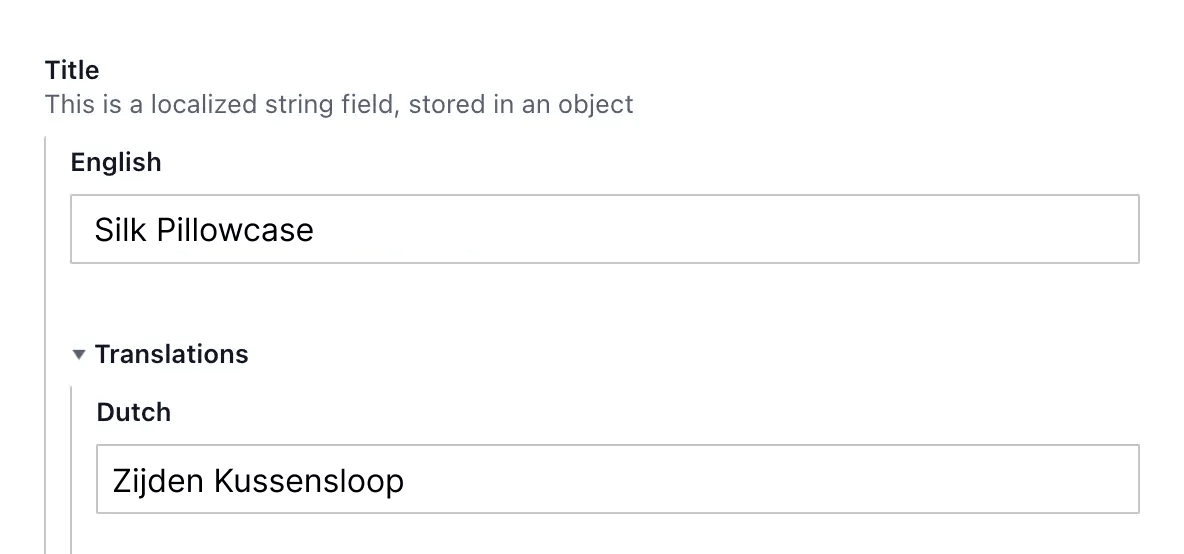The image appears to be a cropped section of a larger page, showcasing a text translation interface. At the top of the image, the word "Title" is displayed in bold black text. Directly below this, in light gray text, it reads "This is a localized string field stored in an object."

Following this, the word "English" is positioned without any surrounding box. Beneath "English" is a text box containing the phrase "silk pillowcase." Directly under this text box is the word "Translations," accompanied by an arrow pointing downward.

Below the arrow, the word "Dutch" is presented. Another text box under "Dutch" contains the Dutch translation "Zijs Den Klessenslap." Throughout the image, all text is black except for the second line that reads "This is a localized string field stored in an object," which is in light gray.

On the far left side of the image, a vertical line runs from the bottom of the second line of text to the bottom edge of the page.